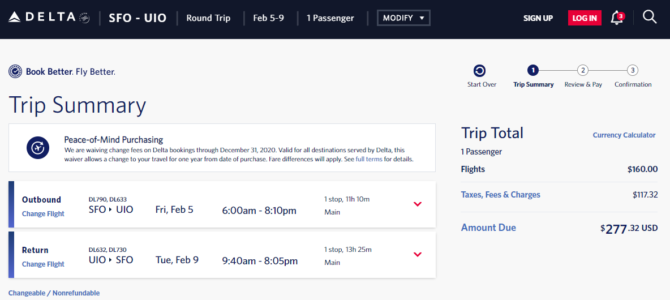The image depicts a detailed screenshot from the Delta Airlines website. The top part of the website features a prominent black navigation bar. On the far left, the Delta logo is displayed in white. Adjacent to the logo, it reads "Delta" followed by "SFO to UIO," indicating a flight route from San Francisco to Quito, Ecuador. Next, it specifies the booking details: "Roundtrip," "February 5 to 9," for "one passenger." There's a "Modify" button allowing changes to the trip settings.

To the right, other options include "Sign Up" and a red "Login" button. A bell icon, highlighted with a red circle containing an exclamation point, signifies alerts. There's also a magnifying glass icon for the search function.

The main body of the webpage is an off-white or pale gray color with blue text. It prominently displays the phrase "Book Better, Fly Better." The trip summary section includes a brief guarantee statement, fine print for transparency, and additional booking details. The outbound flight is detailed as departing from San Francisco (SFO) to Quito (UIO) on Friday, February 5th, from 6:00 AM to 8:10 PM, also showing the total flight duration. There is an option to change the flight, indicated by a red drop-down arrow.

Similarly, the return flight is scheduled for Tuesday, February 9th, from 9:40 AM to 8:05 PM. This segment also includes a change option with a drop-down arrow for more details.

To the right side of the screen, the total trip cost is highlighted under "Trip Total," alongside a currency calculator link. The breakdown reveals the base fare as $160 USD, with additional taxes, fees, and charges, bringing the total amount due to $277.32 USD.